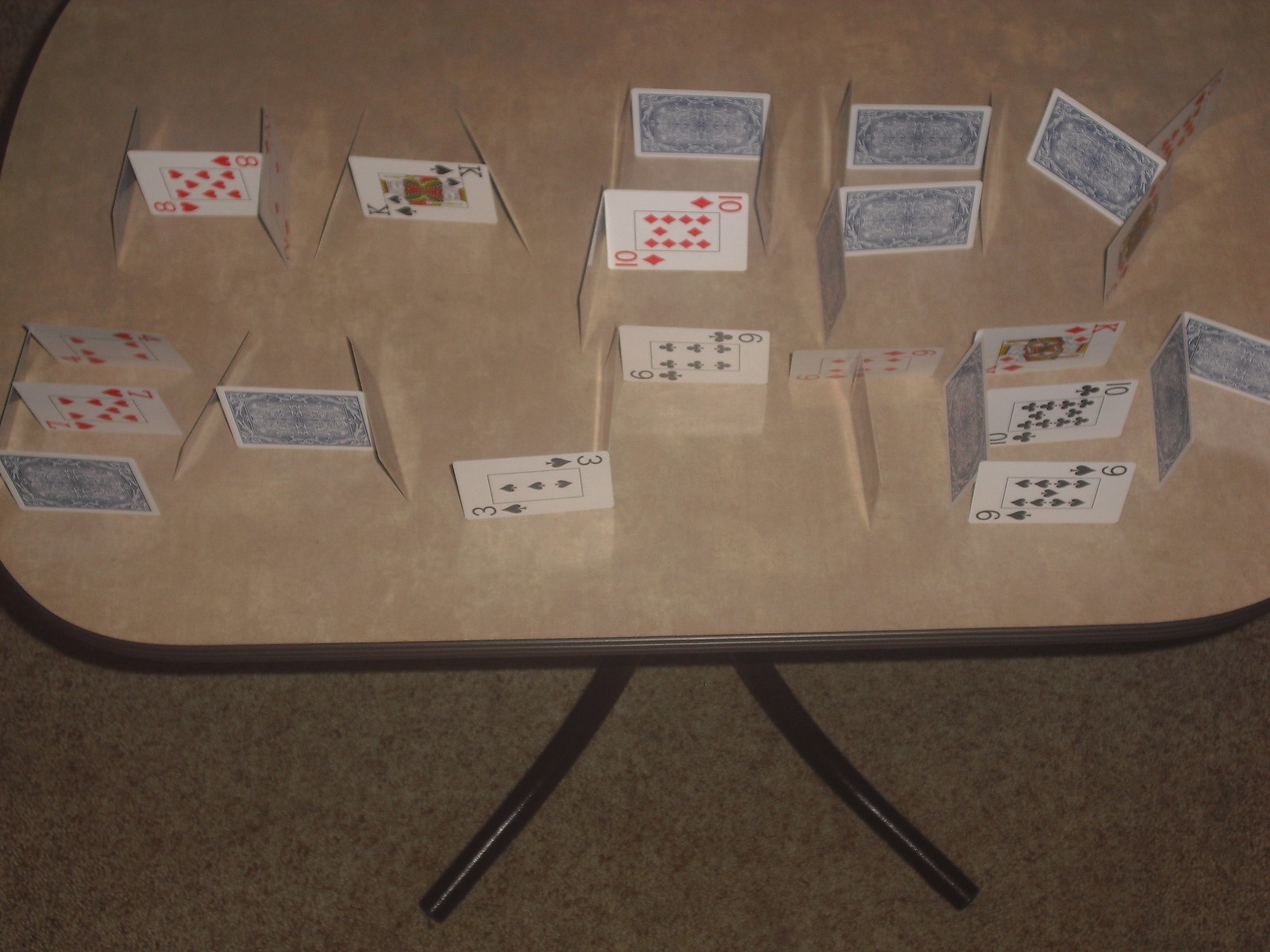In this low-resolution, low-contrast photograph taken in dim lighting, the focal point is an aged table with a faux wood Formica top encased in a dark brown metal band, featuring metal legs that rest upon a thin, brown-gray carpet. The centerpiece of the image is an intricate arrangement of playing cards, carefully stacked on their edges and meticulously supported by additional cards to remain upright. Among the identifiable face cards are the Eight of Hearts, King of Spades, Ten of Diamonds, Six of Clubs, Three of Spades, Seven of Hearts, Four of Hearts, King of Diamonds, Ten of Clubs, and Nine of Spades. Each card is artfully positioned in various patterns, creating an intricate and delicate structure on the tabletop.